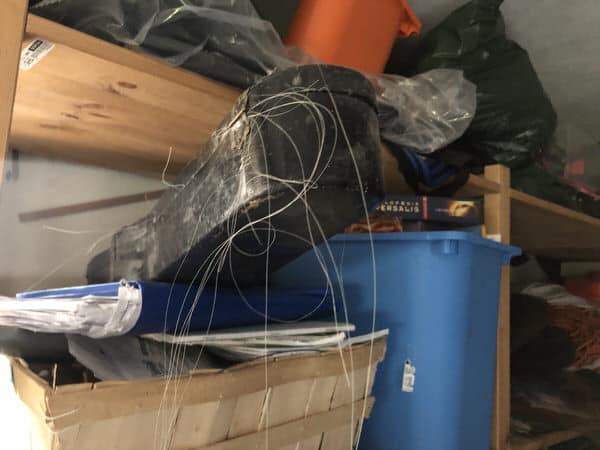A scene of cluttered organization, the image features a woven basket overflowing with loose papers and notebooks on the left side. Beside the basket, a large blue binder, also stuffed with paper, lies beneath a thick, battered guitar or string instrument case. The case, which appears to have endured significant wear and tear, has numerous strings dangling from it, likely guitar strings. Behind this setup stands a trash can of Carolina blue color, containing several discarded books. A table in the background holds various items including sheets of clear plastic wrap, trash bags, and an orange bucket. On the shelf below the table, a collection of towels, rags, and dishcloths is neatly arranged.